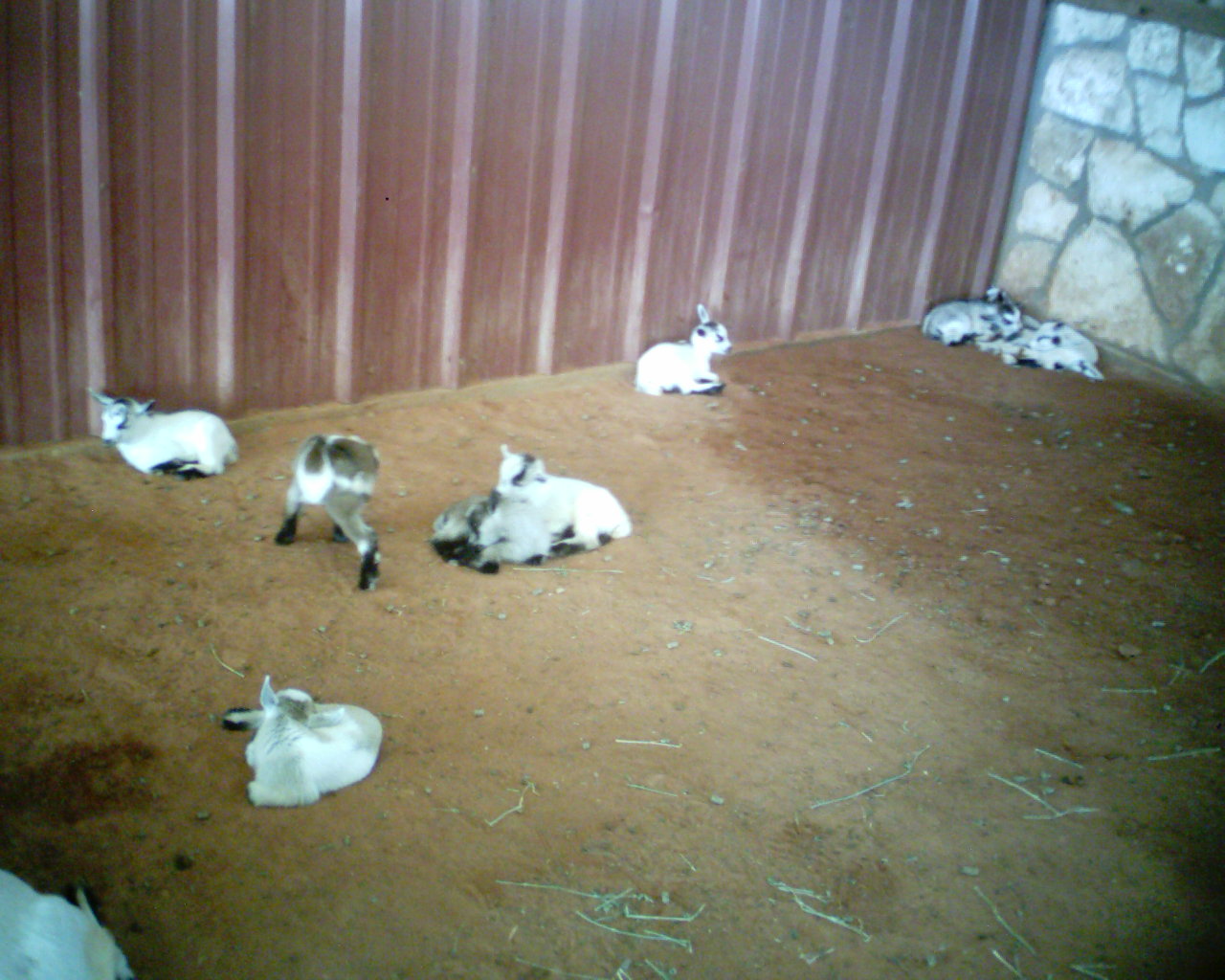This color photograph captures a somewhat out-of-focus corner inside a barn, featuring a group of baby goats scattered across a yellow dirt or cement floor with bits of straw. The far wall on the top left is made of dark brown corrugated metal, while the top right corner displays a geometrically shaped stone or flagstone wall. The floor near the stone wall appears darker, as if recently wet and still drying. Approximately eight to ten baby goats, primarily white with tan legs, heads, ears, and darker feet, are huddling and mingling in various positions. Two baby goats are lying close together in the middle of the image, with one standing in front, seemingly nibbling on something on the ground. In the left foreground, another goat lies down, looking over its shoulder. Several goats are positioned against the back wall like bookends, facing opposite directions, while a small cluster of two or three goats nestle in the back corner where the metal wall meets the stone wall. This charming scene provides a cozy glimpse into the lively and endearing life of baby goats inside the rustic barn.